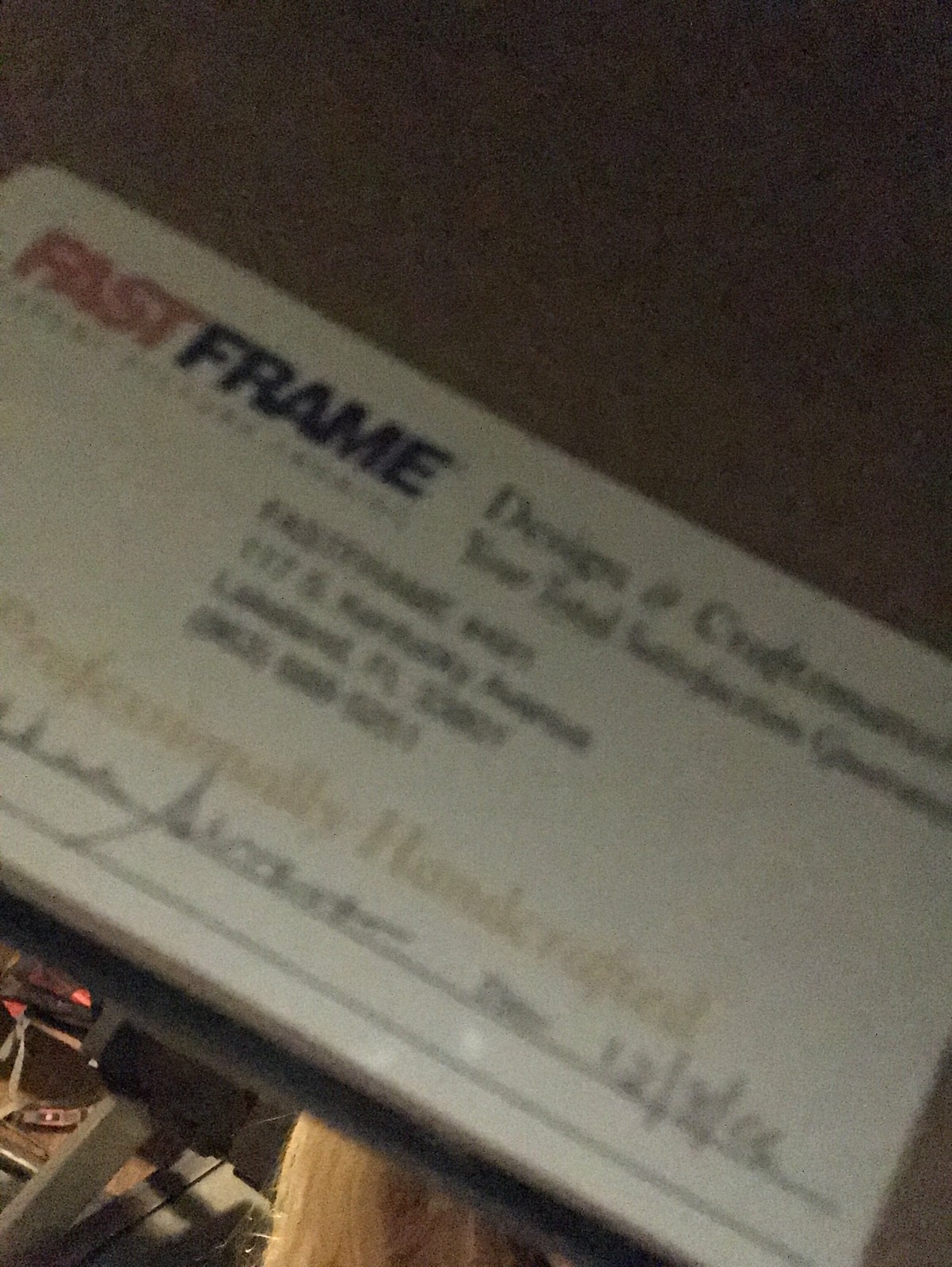This is a detailed close-up image of a business card, which takes up the majority of the frame. Though the writing is somewhat blurry, certain elements can be discerned. In the top left corner, the logo "FASTFRAME" appears, with "FAST" written in bold red capital letters and "FRAME" in blue capitals. Adjacent to the logo, a cursive-style script reads "Design of Craftsmanship." Beneath this, the phrase "YOUR TOTAL SATISFACTION GUARANTEED" is slightly legible despite the blur. Further down, the card features a name and an address, suggesting a location in Florida. Below this address, there is a phone number indicated. At the very bottom of the card, there's a signature and a date, implying that this could also serve as an appointment card in addition to a business card.